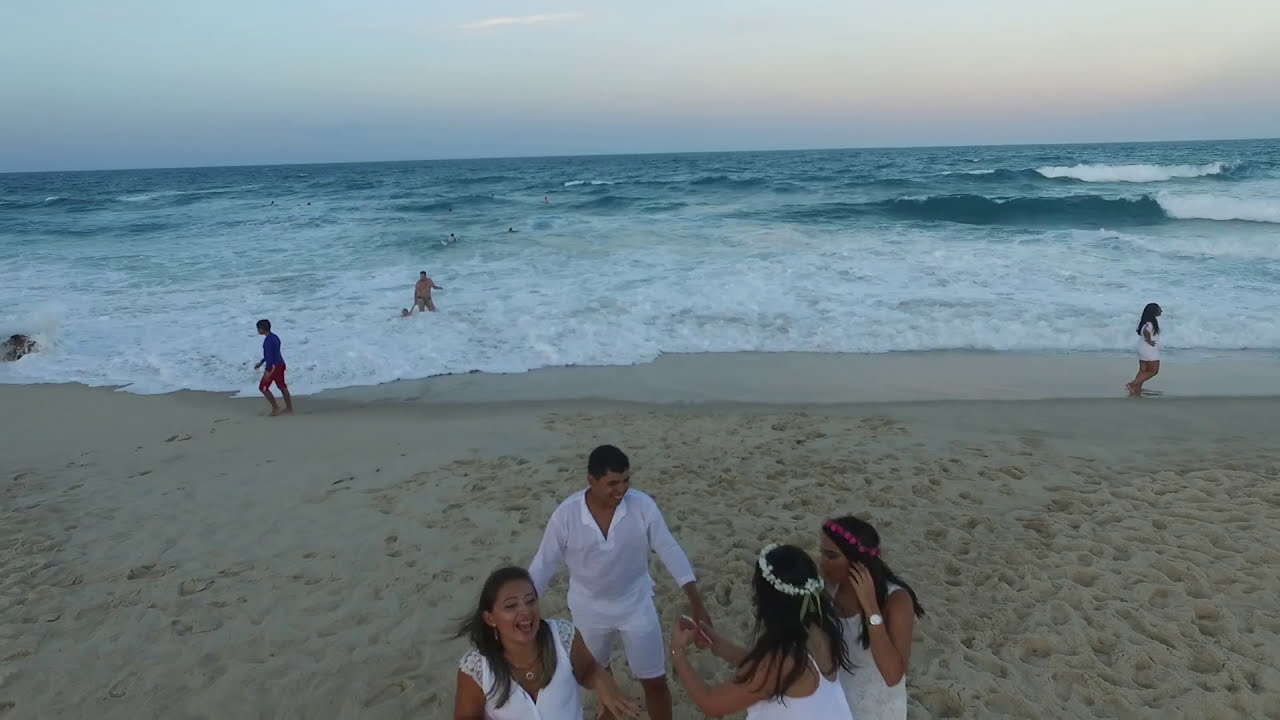This vibrant drone-captured photograph, showcasing a beach gathering from above, vividly details a lively scene set against the backdrop of a setting sun. In the center foreground, a joyous group of four stands out amidst the sandy landscape marked by numerous footprints. The group's focal point is a smiling man in white shorts and a white shirt, characterized by his short dark hair, standing behind three women. All of the women, dressed in white dresses and possessing long dark hair, appear festive and engaged with one another; two wear floral headbands—one with red flowers and the other with white.

Surrounding this central group, the sandy beach extends to meet the lapping waves of the ocean, creating a vibrant mix of tan, blue, and white colors. Several individuals can be seen enjoying the water, swimming or surfing, while others stroll along the shoreline. The distant horizon of this outdoor scene, captured during what appears to be dusk, features a sky transitioning into beautiful hues of pink and purple, framed by scattered clouds. The overall composition is a blend of realism and photographic representationalism, capturing the essence of a joyous outdoor event likely celebrating a party or wedding.